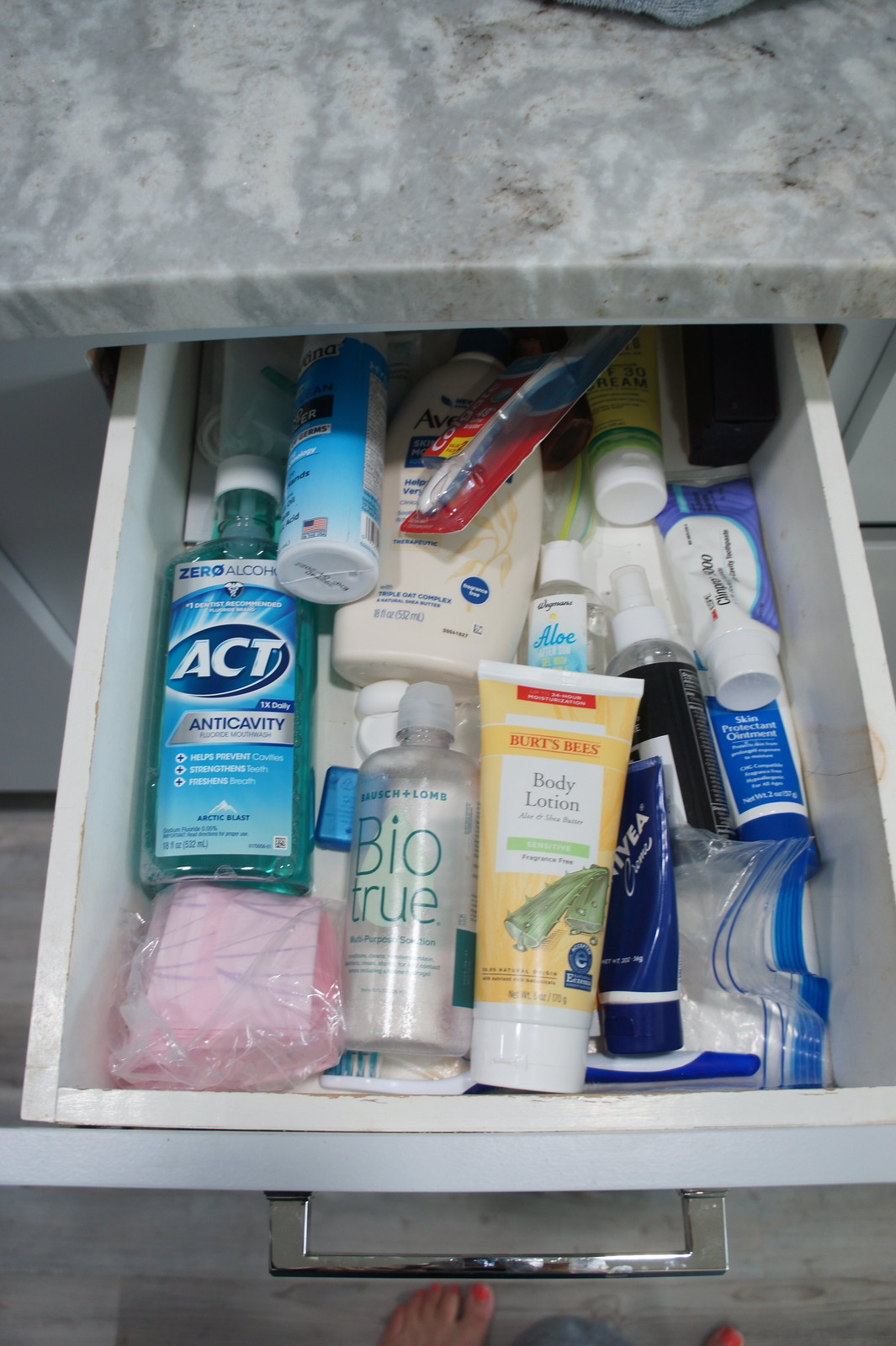This photograph captures the interior of a bathroom, focusing primarily on an open drawer filled with various hygiene products. At the top of the image, stretching from left to right, is a sliver of a gray marble countertop. Below this countertop is the drawer, which features a silver handle at its base. The bottom portion of the image reveals a glimpse of the gray floor, along with a person's bare feet displaying orange painted toenails.

Inside the drawer, a variety of personal care items are neatly arranged. In the top left corner, there is a white tube with a blue label featuring an American flag, possibly a tube of toothpaste. Adjacent to it on the right is a flat, beige-colored bottle labeled "Aveeno." Resting atop this bottle, a red package containing a white toothbrush is visible, with the toothbrush handle protruding from the packaging.

Returning to the left side of the drawer, a blue bottle of mouthwash labeled "ACT Anti-Cavity" is prominently displayed. Moving rightwards from the mouthwash, there is a plastic bag with a pink hue, housing a white square object inside. Further to the right sits a clear bottle of contact solution labeled "BioTrue" in green text. Completing the arrangement on the far right is a yellow bottle with a white label, identified as "Burt's Bees Body Lotion."